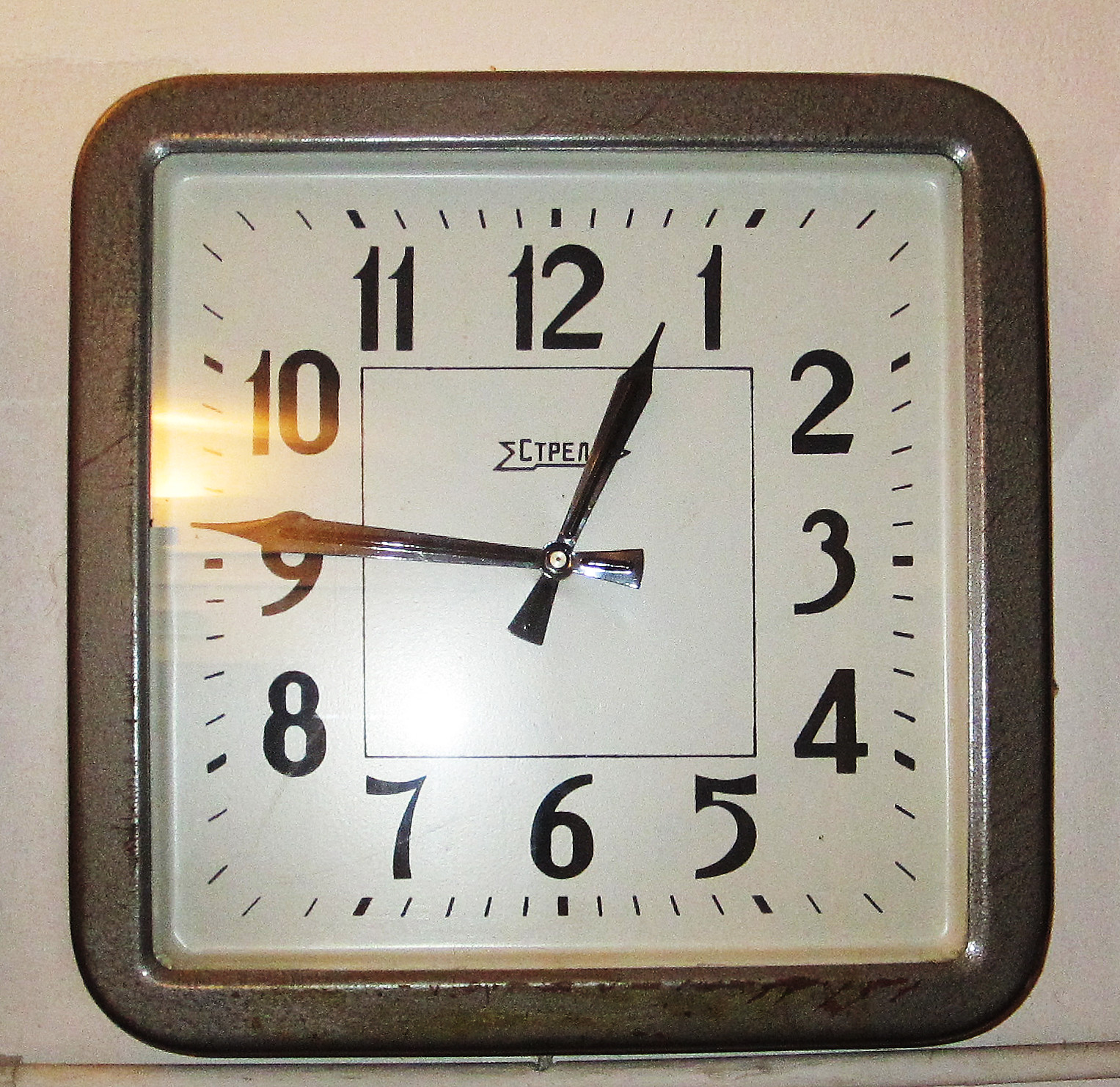An up-close photograph of a square clock with rounded corners against a white background. The metal frame of the clock gleams subtly under the light, while the glass that protects the clock face reflects a gentle shine. The time displayed is 12:46, with the minute and hour hands precisely positioned. The clock's face features bold numbers arranged around a central square design, adding a touch of elegance. Just below the hour hand, the brand name of the clock is faintly visible, though slightly obscured.